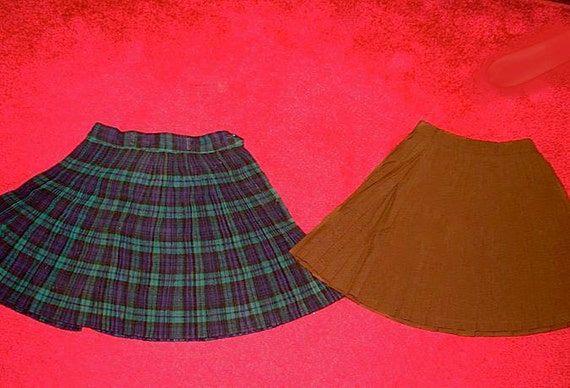This image showcases two skirts laid flat on a red fabric background that seems to be irregular in texture, with some dark areas in the upper corners. On the left side, there's a pleated kilt-style skirt featuring a green and black plaid pattern, reminiscent of a school uniform. The waistband is positioned at the top, and the pleated bottom flares out. The left edge of this skirt is slightly cut off in the photo. To the right, partially overlapping the plaid skirt, is a plain brown skirt, unpleated and straightforward in design. Though this skirt is also partially cut off on the right side of the image, you can see most of it, with its waistband at the top and the skirt flaring out at the bottom, similar to the plaid one.